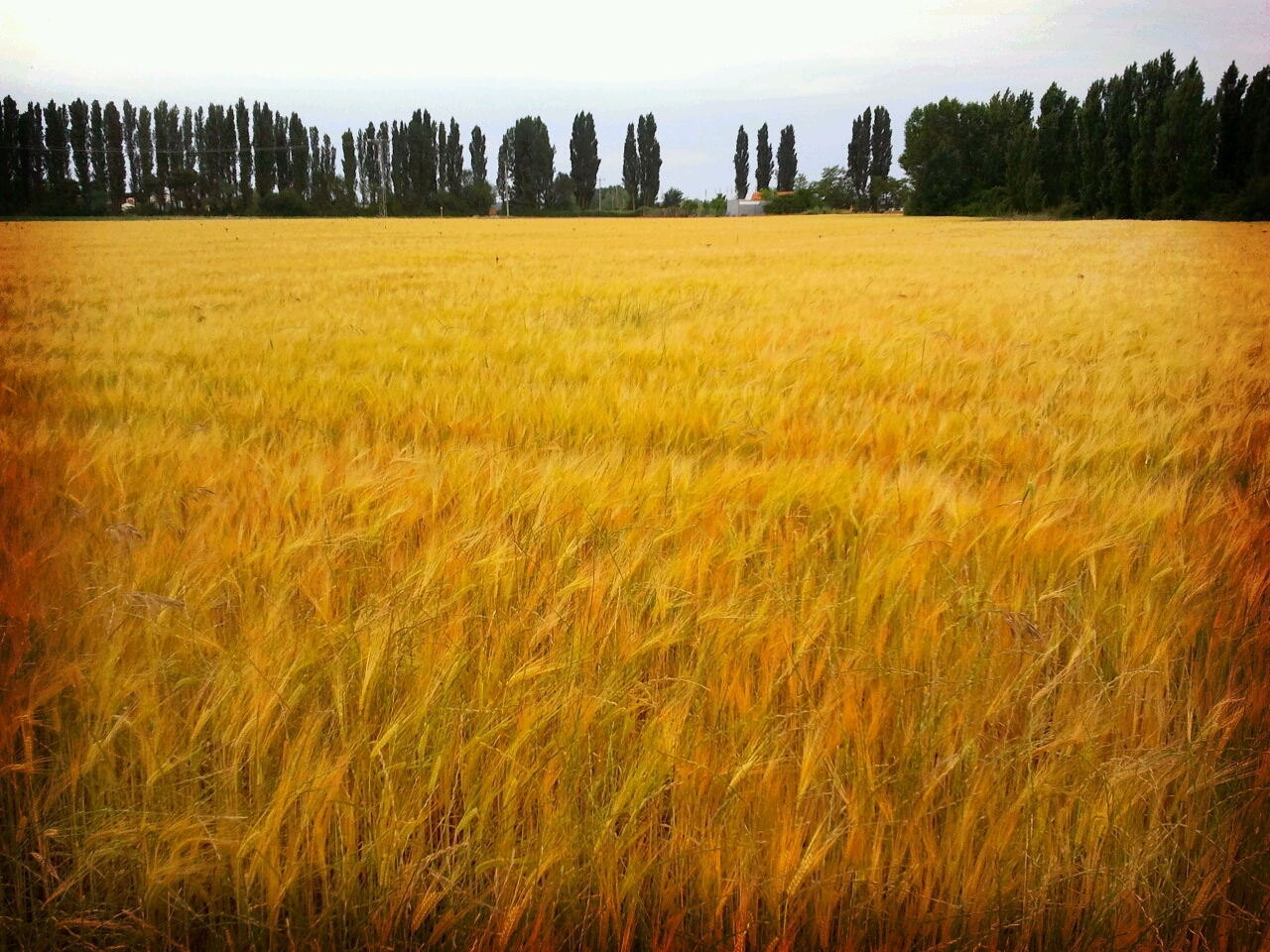The photograph depicts an expansive field of golden wheat grass that stretches across the entirety of the landscape. The vibrant hues of yellowish-green and amber grass dominate the foreground. In the distance, a row of tall, slender trees, including cypress and pine, forms a natural boundary along the horizon. These trees are predominantly dark green and appear to be planted to mark a property line. A white building, possibly a house, stands prominently near the center, with additional structures partially visible to the left. The sky overhead is predominantly blue with streaks of white clouds, indicating a sunny day with some cloud cover. The image, taken from a vantage point two to three feet above the grass, captures the serene beauty of the scene in photographic realism, with slightly darker tones around the bottom edges.